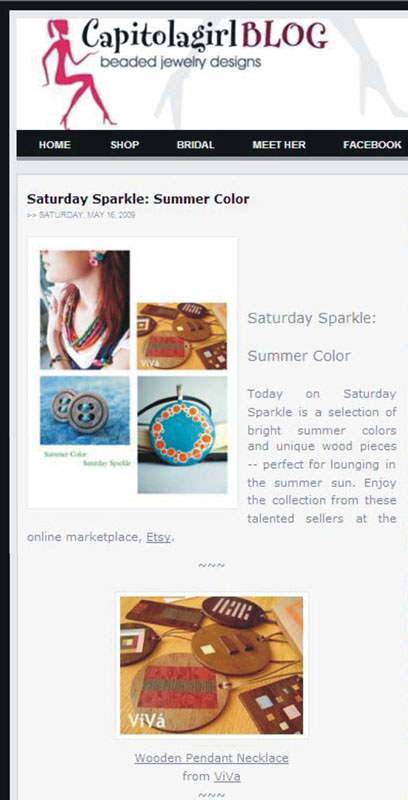The image is a detailed screenshot of a blog website titled "Capital Girl Blog, Beaded Jewelry Designs." At the top of the page, there's an illustrated stick woman sitting and raising her hand next to the title. This indicates the blog likely advertises or discusses beaded jewelry designs, possibly for sale. The header has five navigation options: Home, Shop, Bridal, Meet Her, and Facebook, likely leading to different sections of the site.

Below the header, a section titled "Saturday Sparkle Summer Color" showcases a selection of bright summer-colored beads and unique wooden pendants. There are four images in this section featuring various jewelry pieces, described as perfect for lounging in the summer sun. The text encourages readers to enjoy the collection from talented sellers on Etsy. Additionally, there's a final image at the bottom showing a wooden pendant necklace with intricate designs, emphasizing the unique and handcrafted nature of the items. The page also includes a date, indicating the post was made on Saturday, May 16, 2009. This overall layout suggests a visually appealing, internet-oriented platform promoting handmade beaded jewelry.